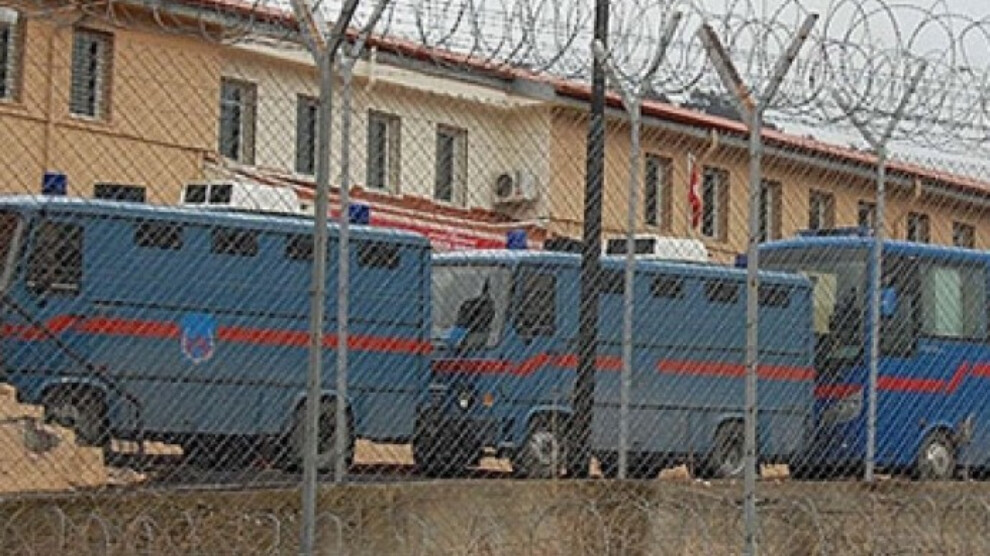The color photograph captures a scene dominated by a chain-link fence topped with a series of menacing barbed wire loops. In the foreground, this imposing barrier suggests a high-security area. Beyond the fence, three prominent vehicles - two large trucks and a bus - are aligned, all uniformly painted a dark blue with a distinctive red stripe along their sides. An official-looking badge is barely discernible on at least one of the vehicles, hinting at their function. The vehicles, parked closely together, have flat fronts and appear designed for transporting prisoners, echoing the security theme. Behind these vehicles stands a nondescript beige building with several windows and a possible Spanish-style roof. The sky, overcast and grey, adds to the somber atmosphere. The ground in the image consists of brown soil, completing the overall stark and secure environment, likely that of a maximum-security prison or similar facility.